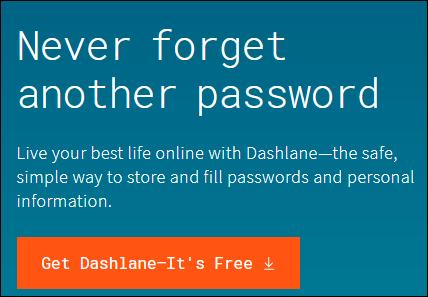The image features a gradient blue background that transitions from dark blue at the top to a lighter blue at the bottom. Central to the image, a message is displayed in light blue text: "Never forget another password. Live your best life online with Dashlane." Below this, another line in similar light blue text reads: "The safe, simple way to store and fill passwords and personal information."

Prominently positioned underneath this text is a large, bright orange button with white, bold letters that say, "Get Dashlane. It's free." To emphasize the call to action, the button features a down arrow with an underlining line below the text.

The overall design clearly communicates the benefits of using Dashlane for password management and invites viewers to download the app with a visually striking and easy-to-understand call to action.